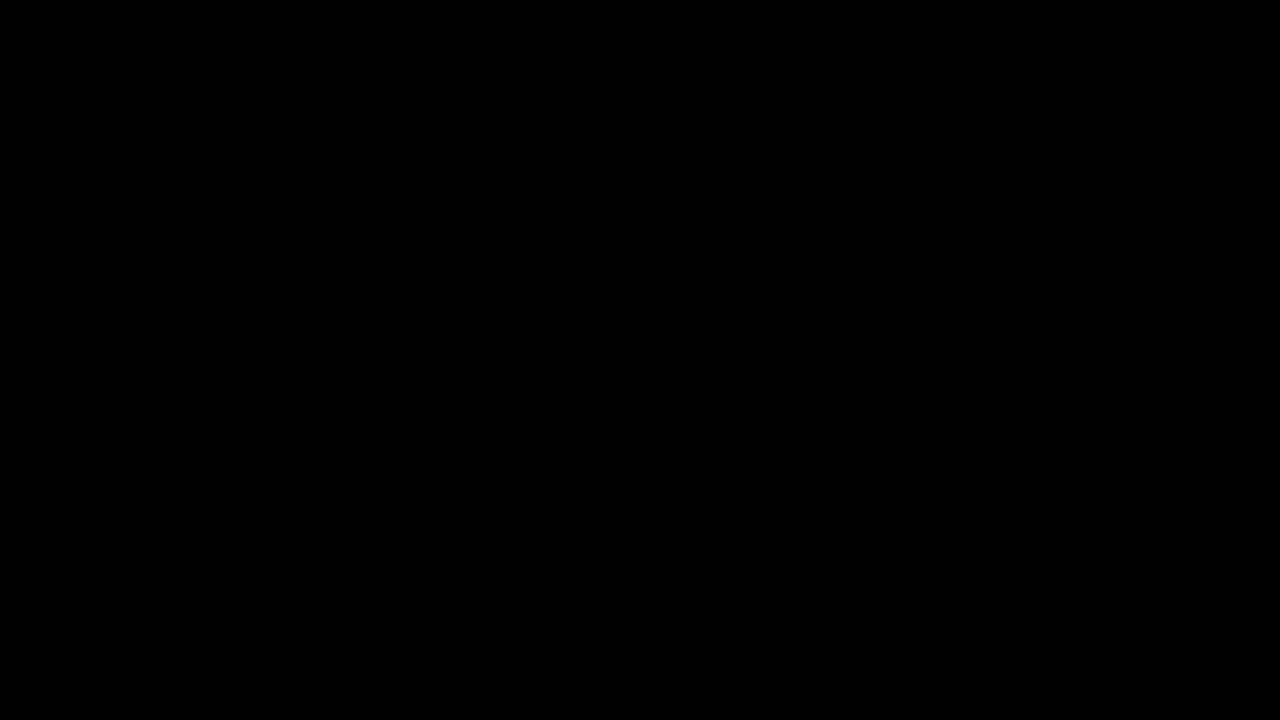The image is a completely black rectangular shape, wider than it is tall, reminiscent of a void. There are no objects, text, or any other visual elements present in the frame. The only visible color is black, which dominates the entire picture, creating an impression of total darkness or a possible glitch.